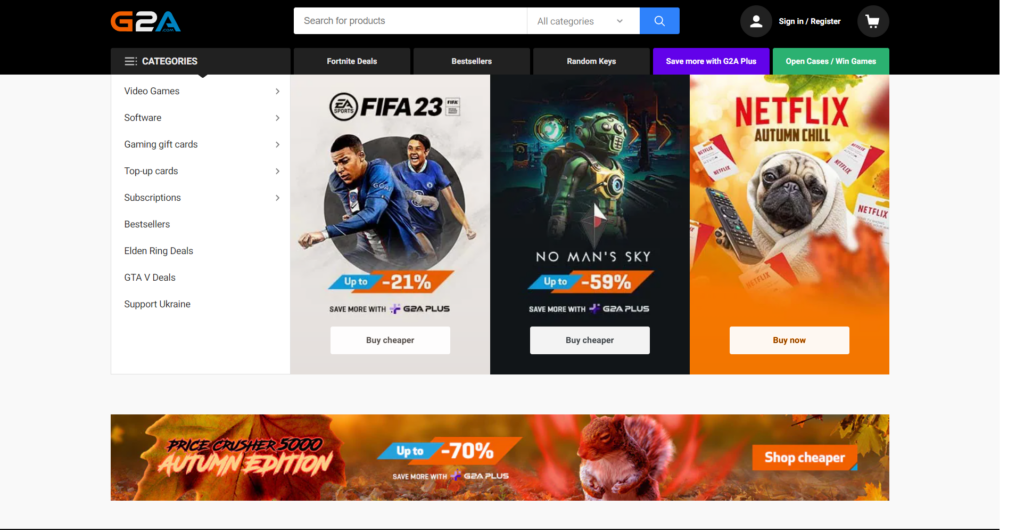Screenshot of a gaming website "G2A" featuring various product categories and promotional offers. The website's header is dark gray, with a search field labeled "Search for products" and a blue search button. Links for "Sign In," "Register," "Shop in Cart," and various product categories like "Fortnite deals," "Bestsellers," "Random Keys," and "Save More with G2A+" are displayed under the header, with tabs in light to medium gray and purple, and a green tab hinting at gaming rewards.

The "Categories" section lists options such as "Video Game Software," "Gaming Gift Cards," "Top-Up Cards," "Subscriptions," "Bestsellers," "Elden Ring Deals," "GTA V Deals," and "Support Ukraine." Adjacent to this is promotional content, including a green cover art for "FIFA 23" offering up to 21% off with a "Buy Cheaper" button, and art for "No Man's Sky" featuring a green robot with an offer up to 59% off, alongside a similar "Buy Cheaper" button. Lastly, a "Netflix Autumn Chill" promotion with an image of a pug wrapped in a towel, featuring a remote control and a "Buy Now" button.

At the bottom is the "Price Crusher 5000, Autumn Edition," indicating savings of up to 70% with an illustration of a squirrel emitting power beacons and an invitation to "Shop Cheaper."